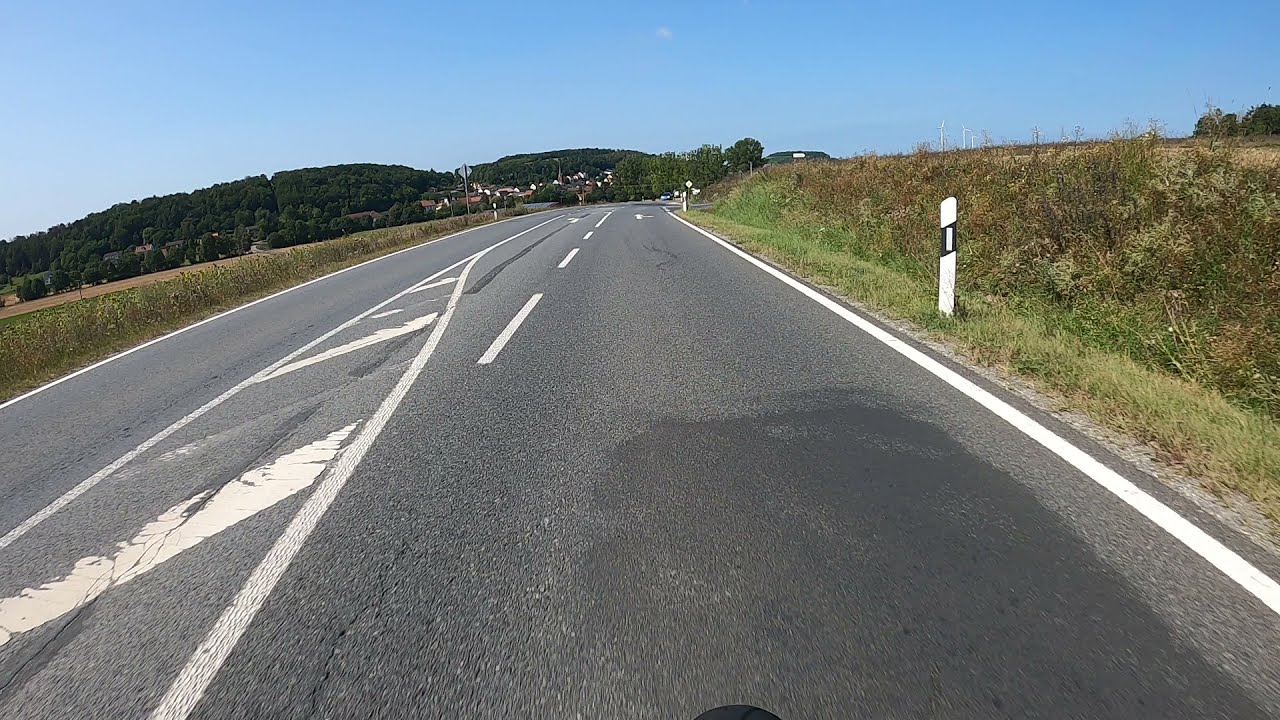This detailed photograph showcases a green asphalt road that stretches ahead and gently curves to the right. The road features several white line dividers, including solid lines on both sides and a combination of solid and broken lines in the center, indicating lane separation. A directional arrow provides an option to turn left further ahead. On either side of the road, the terrain is lush with grass and plants, while black and white posts mark the road's boundaries. In the distance, a hill covered with dense trees adds to the picturesque scenery, hinting at a nearby town nestled within this verdant landscape. Above, the sky is a clear, bright blue, free of clouds, enhancing the serene and vibrant atmosphere of the scene.